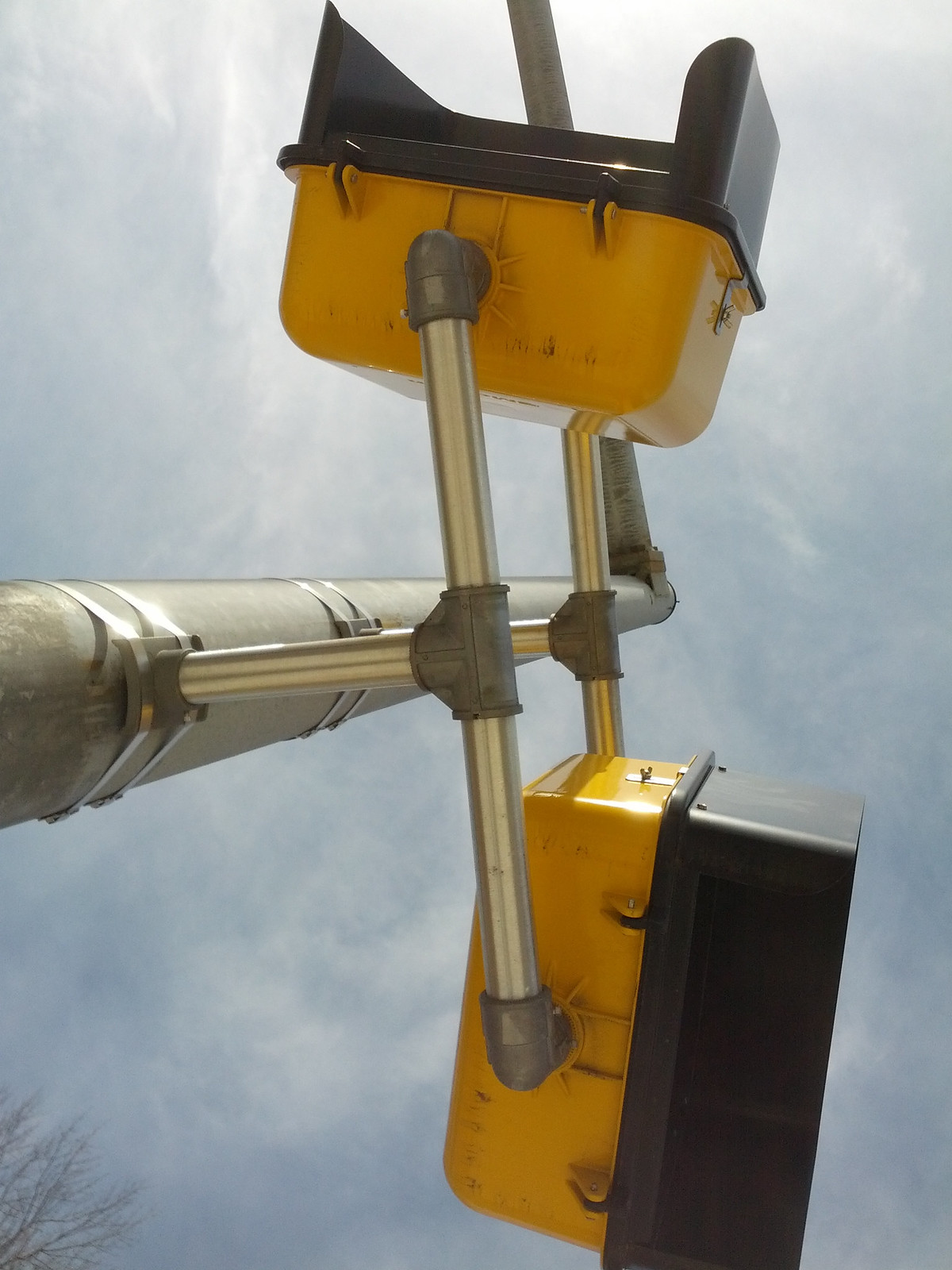This outdoor color photograph, taken in bright daylight, captures a detailed, upward-looking view of a street lamp and accompanying pedestrian signals. The shot is oriented vertically, with the long side of the rectangle stretching from top to bottom, emphasizing an almost vertical perspective. The main street pole enters the frame from the left and extends towards the background, ending about two-thirds into the photograph. Horizontal bracketing supports two pedestrian signal boxes: one positioned towards the top of the image and the other facing right.

The signal box at the top features an orange background with a plastic shroud, pointing upwards. The other signal box, similarly constructed, has a yellow body and a black hood, facing to the right. Both boxes resemble typical walk or don't walk signs, securely attached to the pole with chrome-metal handles. The background showcases a light blue, hazy sky with hints of white, and a tree's foliage entering from the lower left corner of the frame. The photograph is in sharp focus with no visible text or words.